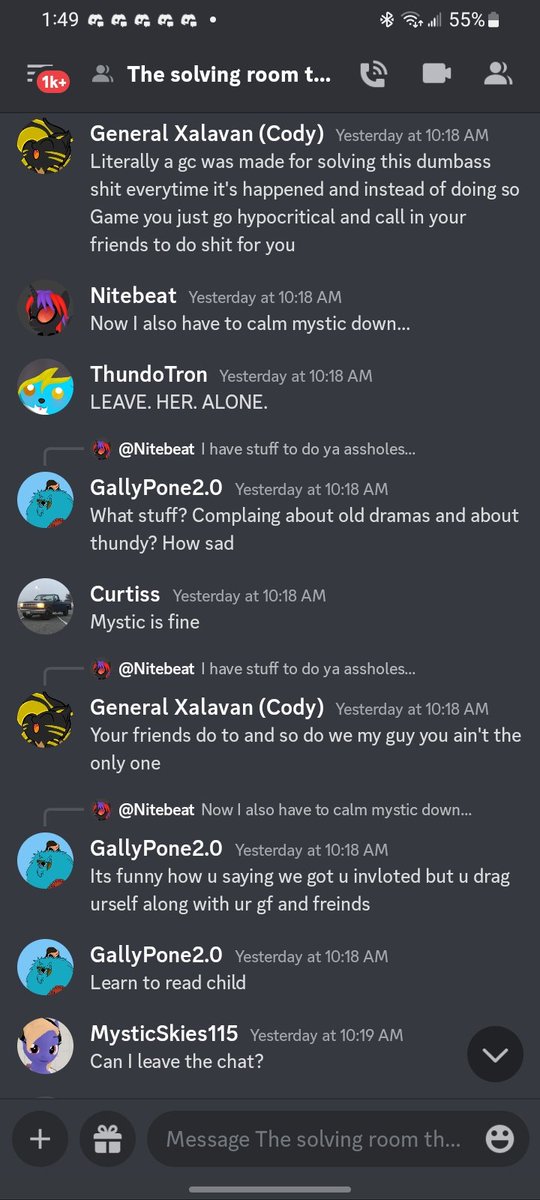This image is a screenshot captured from a cell phone, depicting an intense and somewhat chaotic conversation happening within a chatroom titled "The Solving Room...". The background is entirely black, while the text appears in contrasting white and gray fonts, enhancing readability.

On the left side of the image are small profile pictures representing the participants, with their messages displayed to the right. At the top, General Kalbazan drily remarks, "Literally, a GC was made for solving this dumb ass shit every time it's happened, and instead of doing so, game, you just go hypocritical and call in your friends to do shit for you." Following this, another user comments, "Now, I also have to calm Mystic down..."

The conversation escalates as Thundotron interjects, "Leave her alone." Meanwhile, Gallypon2.0 quips, "What stuff? Complaining about old dramas and about Thundie, how sad." In response to the brewing tension, Curtis reassures, "Mystic is fine."

General Xavin then counters, "Your friends do too, and so do we, my guy. You ain't the only one." The debate continues with a participant pointing out, "It's funny how you say, and we got you involided, but you drag yourself along with your GF and friends," followed by a curt retort, "Learn to read, child."

The discord reaches a peak with one user exclaiming, "Can I leave the chat?" encapsulating the drama and intensity of the digital altercation.